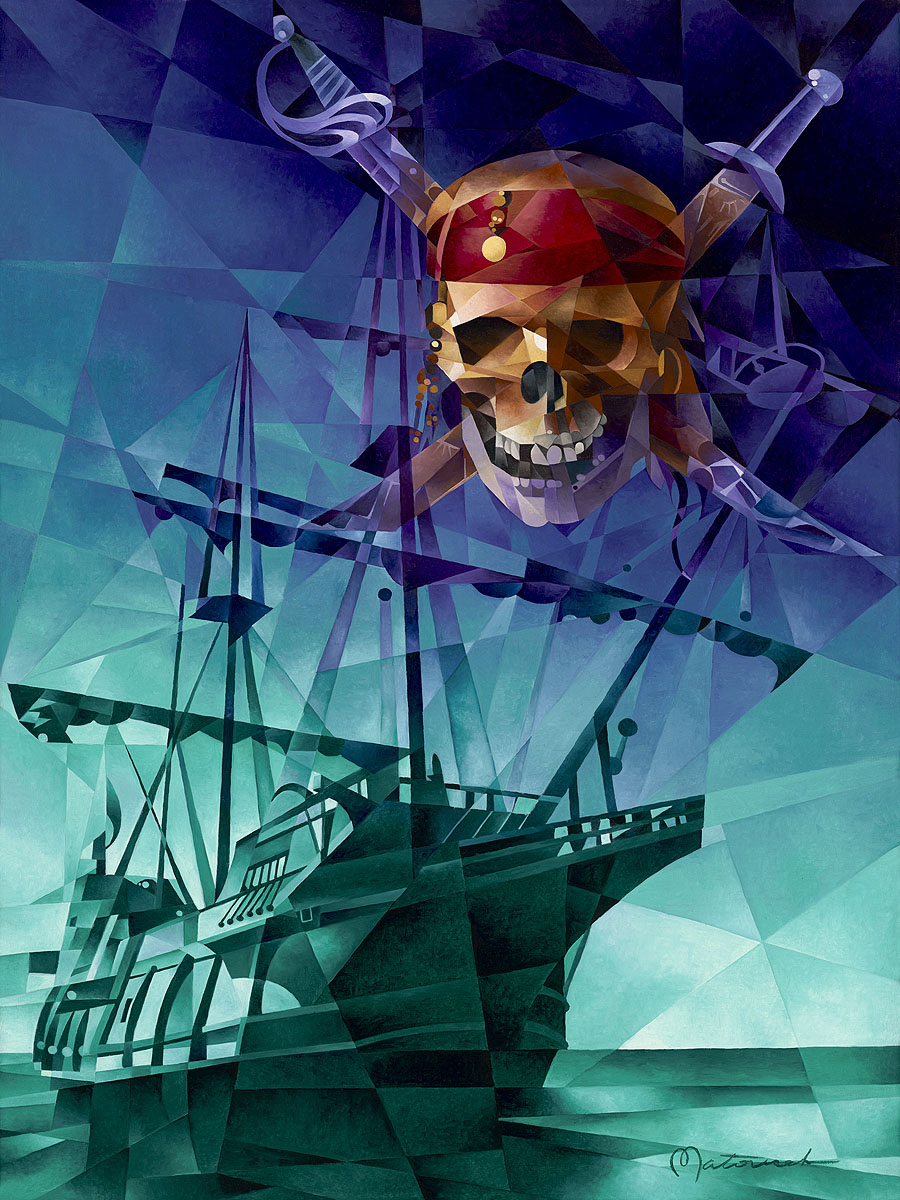This digital artwork features an abstract yet recognizable design with a predominant pixelated, prismatic pattern composed of diamonds, triangles, and other shapes. The upper portion of the image is shaded in dark purple, blending seamlessly into an aquamarine hue towards the bottom. In the upper right corner, set against the purple background, is a detailed pirate skull adorned with a red bandana and decorated with two beads and a gold coin. The skull, characterized by its brown hue and missing front tooth on the viewer's left, has a purple jawline and two purple swords crossed behind it, forming an X. The bottom left corner showcases a pixelated pirate ship in teal or aquamarine tones, without any visible sails. A signature, possibly reading "M-A-T-O-R-V-E-H," is located in the bottom right-hand corner, indicating the artist's name. Overall, the colorful and intricate patterns give the artwork a unique, abstract quality.